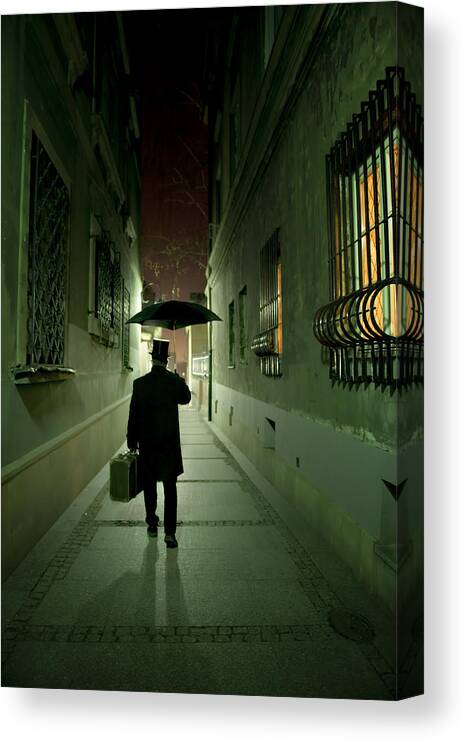The painting on canvas vividly portrays a nighttime scene of a man, dressed in a black suit, black pants, a black hat, and carrying an open umbrella high above his head in his right hand, and a suitcase in his left hand. He is depicted walking down a narrow alleyway with granite sidewalk and brick patterns between each square, towards a light source that is obscured by his figure, casting a long shadow behind him. The alleyway is flanked by two- to three-story buildings with barred windows on both sides. On the right-hand side, some windows are lit, casting light onto the pavement, while the left-hand side windows remain dark. The buildings have a weathered, greenish tone with white accents near the base. The dramatic sky above transitions from black to a darkish red, adding to the eerie, mysterious atmosphere. The image elegantly wraps around the visible side of the canvas, enhancing the three-dimensional effect of the painting.